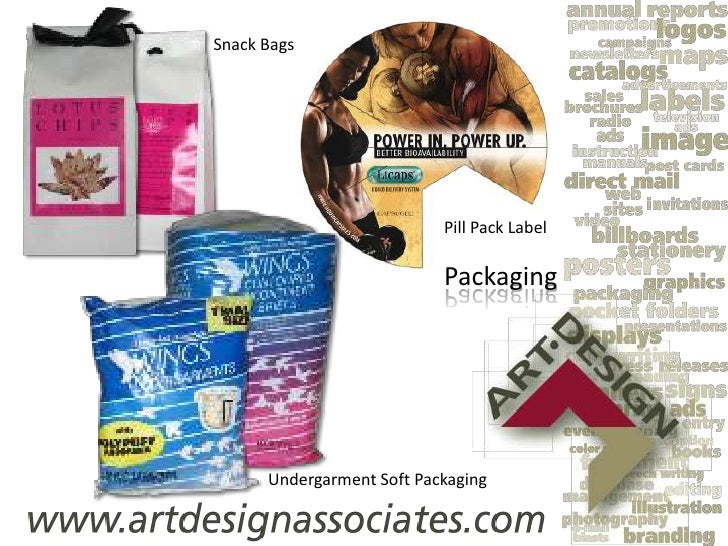The advertisement image showcases a variety of packaging designs and concepts, prominently displaying the branding and product offerings of www.artdesignassociates.com. In the upper right corner, there are several white gift bags with pink labels and black ribbon ties labeled as "snack bags" in black ink. Adjacent to these bags is a circular design featuring the profile of a muscular woman lifting weights, with the text "Power In, Power Up" and "Pill Pack Labeling" beneath it. Toward the lower left center, two overlapping bags are visible; one is blue with white lines, while the larger bag has additional pink lines. These bags are labeled as "Undergarment Soft Packaging." The right half of the image features a column with various overlaid words, such as annual reports, promotion logos, campaigns, and catalogs. At the bottom of this column is a logo for "Art Design." The color palette includes pink, white, blue, black, and other shades, arranged in a somewhat disorganized yet visually appealing manner, effectively highlighting the versatility and creativity of the packaging designs offered.